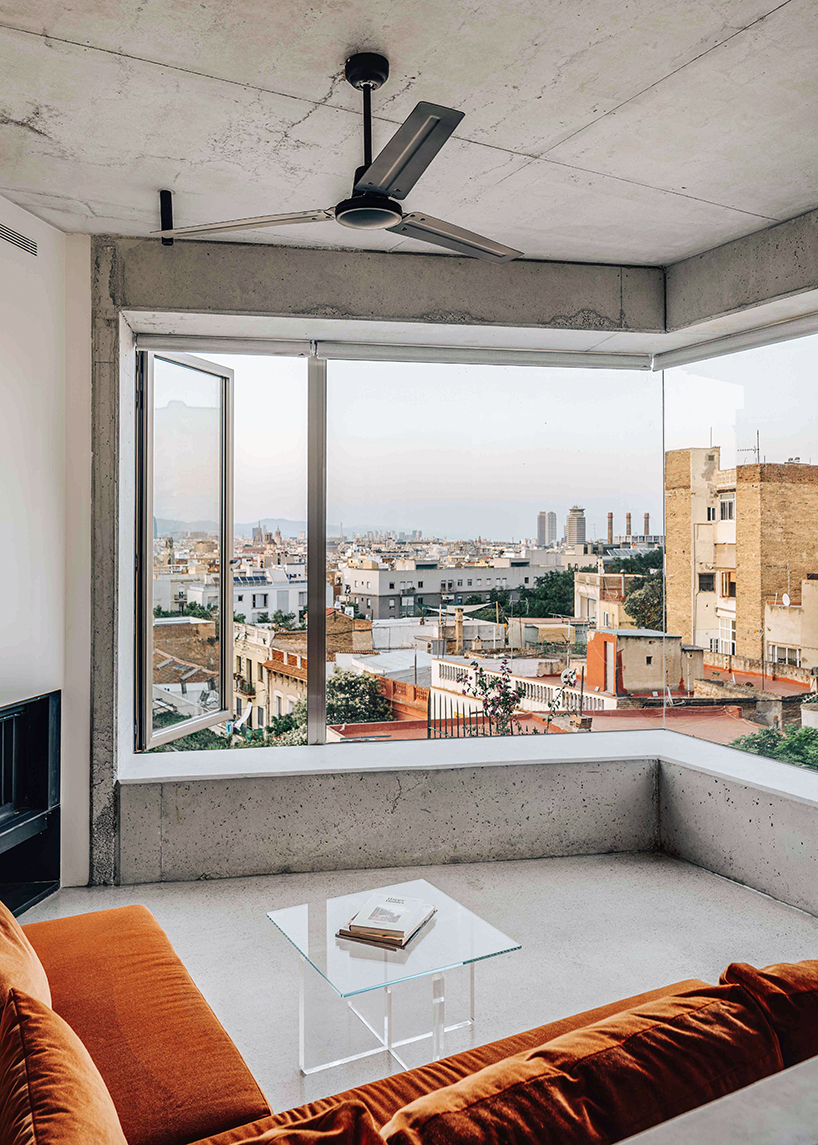The photograph showcases a contemporary, high-floor apartment living room characterized by large, floor-to-ceiling, L-shaped glass windows, cornering two sides of the space. The leftmost panel of the glass window is a crank window that opens outward, allowing an extensive, unobstructed view of a sprawling cityscape comprising multicolored buildings in hues of white, orange, brown, and gray. Some of these buildings have flat roofs and vary in height, with a few towering structures visible in the distance, surrounded by a sky tinged with light blue and pink, indicative of a smoggy day.

Inside the apartment, the decor features a modern aesthetic with a polished concrete floor and ceiling, while the walls, predominantly white, also showcase sections of gray concrete. A rust-colored, L-shaped sectional sofa takes prominence in the seating area, accompanied by a small, square, glass-topped coffee table with a white metal cross-type support, holding two or three books. Adjacent to the sofa, on the left wall, a black-outlined raised fireplace adds to the room's cozy yet minimalist design. Overhead, a black, three-bladed ceiling fan hangs from the marble-patterned ceiling, contributing to the room's airy feel. The overall ambiance of the room is open, uncluttered, and well-lit, emphasizing the expansive urban view through the vast glass windows.